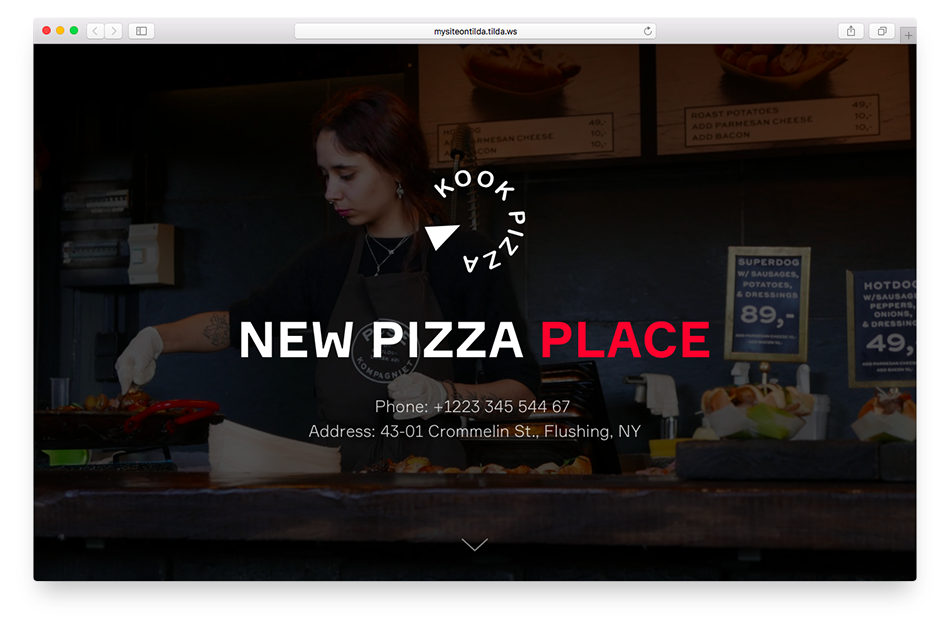Screenshot of the Kook Pizza webpage with browser tabs visible at the top. The webpage features the restaurant's logo, "Kook Pizza," with the letters "K-O-O-K Pizza" arranged in a circular pattern. A white arrow resembling a pizza slice is integrated into the design. Below the logo, the text "New Pizza Place" is displayed, with "New Pizza" in white and "Place" in green. The contact information is provided: "Phone: +1 223 345 5446" and the address listed as "43-01 Crommelin Street, Flushing, New York." In the background, there is a dimmed image of a woman cooking in a skillet. She has black hair, white skin, and is wearing a black shirt or apron along with white gloves.